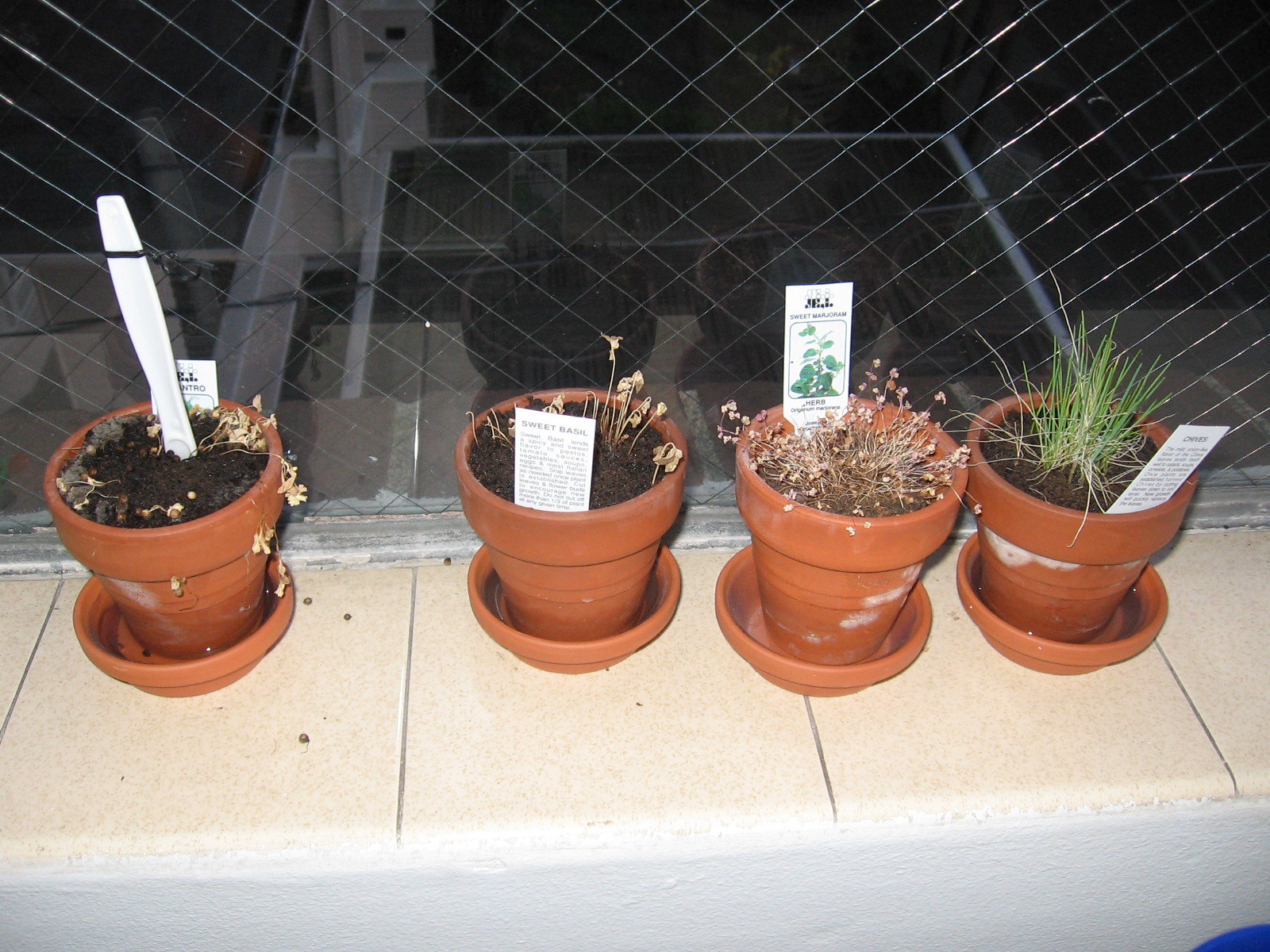A detailed photograph captures four terracotta plant pots, each paired with a matching tray, lined up on a light tan tile ledge against a backdrop of wire-reinforced glass. The scene appears to be at night, suggested by the reflection in the glass and the absence of daylight. Starting from the left, the first pot contains dark soil with a dead cilantro plant. A dried leaf hangs over the side, and a makeshift support, possibly a plastic knife handle, stands upright with a black tie on it, next to a partially visible plant marker. The second pot houses a dried sweet basil plant with light brown stems, labeled by a prominent white tag stuck into the soil. The third pot features a withered sweet marjoram plant with low, dry foliage and a white marker indicating its name. The fourth and final pot contains the only thriving plant in the group, green chives, which are a few inches tall, marked by a white tag at the front. The wire mesh behind the pots and the faint reflections suggest the pots sit on an interior windowsill, possibly near a kitchen sink.